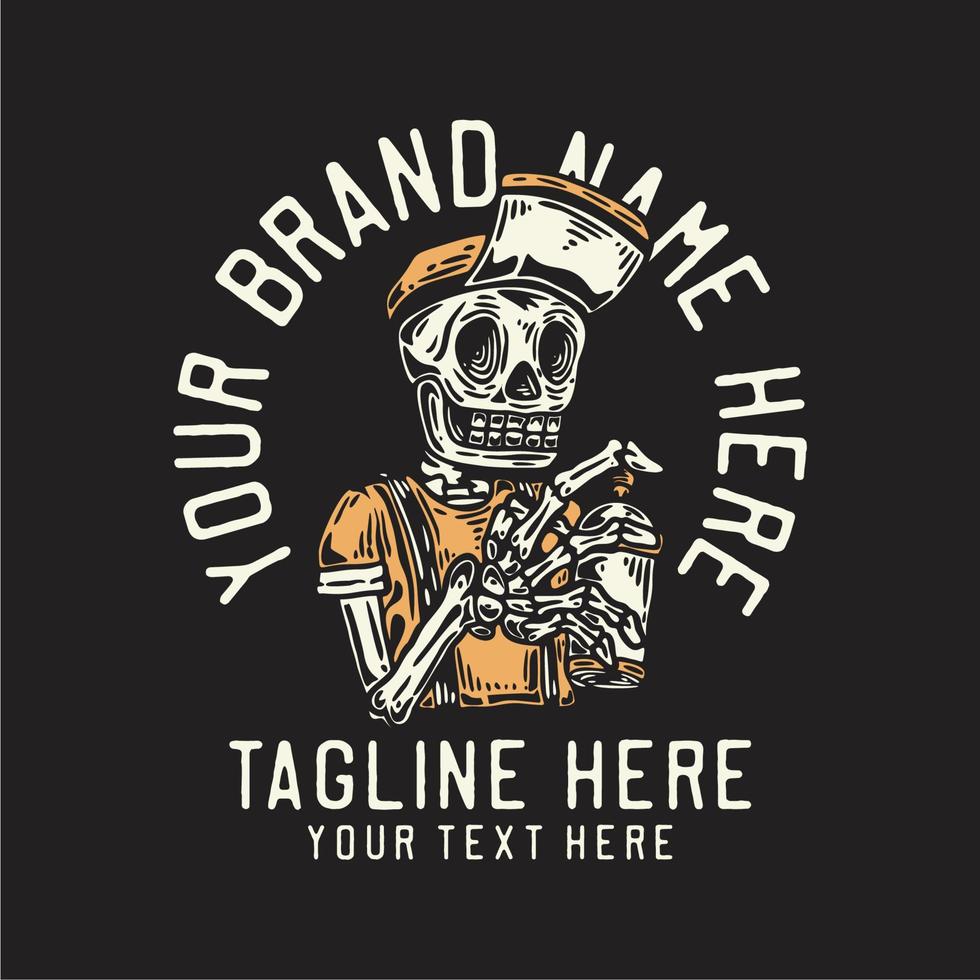This image is a detailed mock-up template designed for businesses to customize with their own branding. The central figure is a smiling skeleton wearing an orange baseball cap with the bill turned up, an orange short-sleeve shirt, and black suspenders. The skeleton's facial features detail drilled-out eye holes with spirals and pronounced teeth. In its bony hand, it holds a spray can. Surrounding the skeleton in a circular layout is the placeholder text "Your Brand Name Here" written at the top, with "Tagline Here" directly below it, and "Your Text Here" underneath the tagline, all in white text. This template seems to be intended for creating personalized t-shirts or logos, and it provides space for a business to insert their brand name, tagline, and custom text.